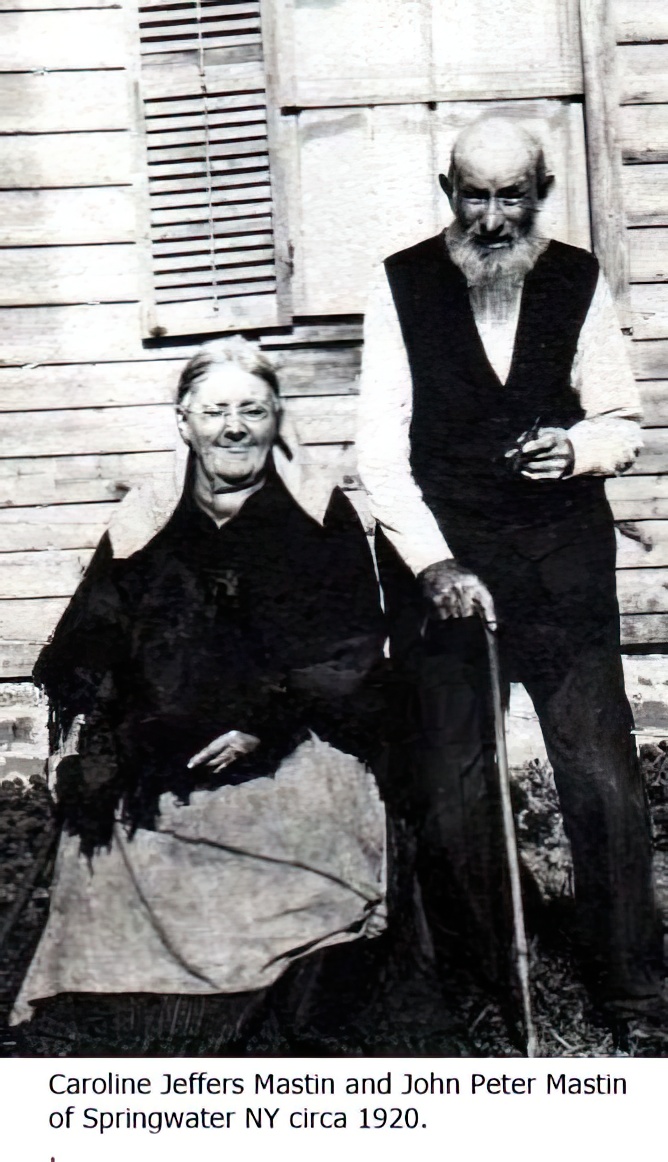The black and white photograph from circa 1920 captures Caroline Jeffers Mastin and Joe Peter Mastin in front of their wooden, unpainted house in Springwater, New York. The house, featuring storm shutters and white curtains visible through the windows, is bathed in natural daylight, illuminating the scene. Caroline Jeffers Mastin is seated in a chair, donning a long-sleeve coat over a skirt, a white shawl draped over her shoulders, and metallic-rimmed glasses. Her hair is tied back, and she sits calmly. To her right stands Joe Peter Mastin, leaning on a wooden cane with his right hand. He is dressed in black pants, black shoes, a vest over a long-sleeve button-up shirt, and has a bushy white beard and a bald head. In his left hand, he holds a smoking pipe. The photograph is detailed with a white banner at the bottom, bearing the caption in black text: "Caroline Jeffers Mastin and Joe Peter Mastin of Springwater, New York, circa 1920."